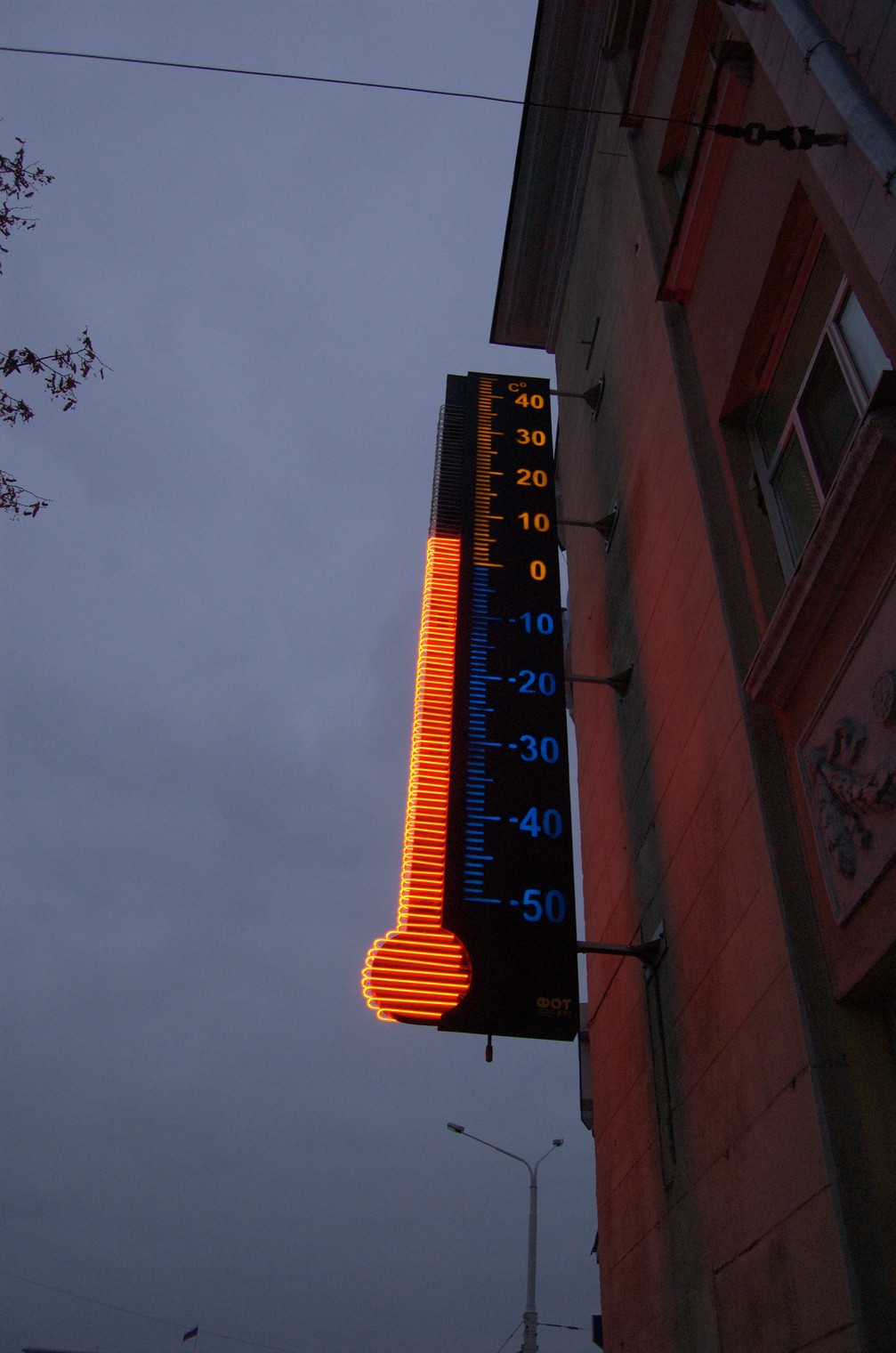This photograph, oriented vertically, captures the exterior of a large stone building during either the early morning or late evening, as suggested by the dim, gray, and cloudy sky. The building, constructed from brown-colored stone and standing at least three stories high, occupies the right-hand side of the image. The left-hand side reveals the overcast sky, accented by a small cluster of tree leaves in the top left corner. Additionally, a horizontal wire is visible at the top, connecting to the building. 

Prominently attached to the side of the building is a tall, slender, illuminated sign designed to resemble a thermometer, indicating the current temperature. The sign, with blue numerals denoting subzero temperatures and red numerals for warmer readings, ranges from -50 degrees Celsius at the bottom to 40 degrees Celsius at the top. The illuminated red fluid marker shows the temperature as 5 degrees Celsius, providing a clear and functional element to the imposing stone facade.